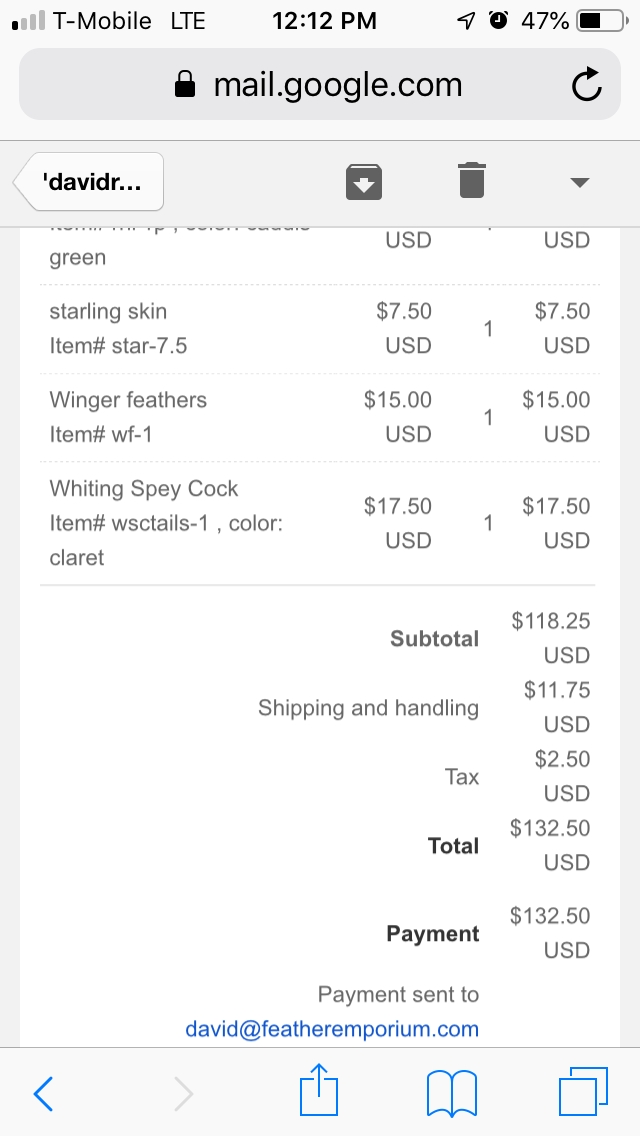The image depicts a screenshot of an email containing a receipt, viewed on a mobile device, likely a phone or tablet. At the top left corner of the screen, the status bar shows "T-Mobile LTE" with a signal strength icon at 104 bars. Centered at the top, the time is displayed as 12:12 p.m., and the top right corner includes icons for directional navigation, a clock, and a battery indicator showing 47% charge.

Below this, there is a search bar featuring a lock icon and the URL "mail.google.com," accompanied by a refresh button. The email appears to be from "David R." and includes options for downloading or deleting the message via icons next to the sender's name.

The main body of the email includes a white section detailing the receipt of an order from Feather Emporium. The itemized list specifies:

1. **Star Wing Skin Item** (Star 7.5) - $7.50 USD
2. **Wing Feathers** (Item Number WF-1) - 1 unit at $15.00 USD
3. **Whiting Spey Cock** (Item WSC Tails 1, Color Claret) - $17.50 USD 

The subtotal comes to $118.25 USD, with shipping and handling adding $11.75 USD, and tax contributing an additional $2.50 USD. The total amount is listed as $132.50 USD, which has been duly paid. The payment recipient is noted as "david@featheremporium.com."

Additional icons, including a back arrow, an upload symbol, and a double rectangle for multitasking, are visible below the total payment information.